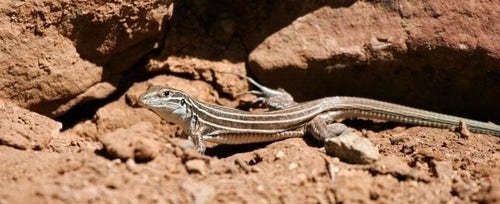This full-color, horizontally rectangular image was taken outdoors on a sunny day in a warm, desert-like climate. The background consists mostly of dirt, pebbles, and large, nondescript brown rocks that cast subtle shadows. The foreground features an earthy, rocky terrain sprinkled with small rocks and tufts of grass. The central focus of the image is a dark green-gray lizard with a long tail and distinctive brown and white stripes. The lizard is in profile, facing left, showcasing its textured, ribbed white belly. The photo is zoomed in, emphasizing the lizard's details while capturing only a small area of its immediate environment.